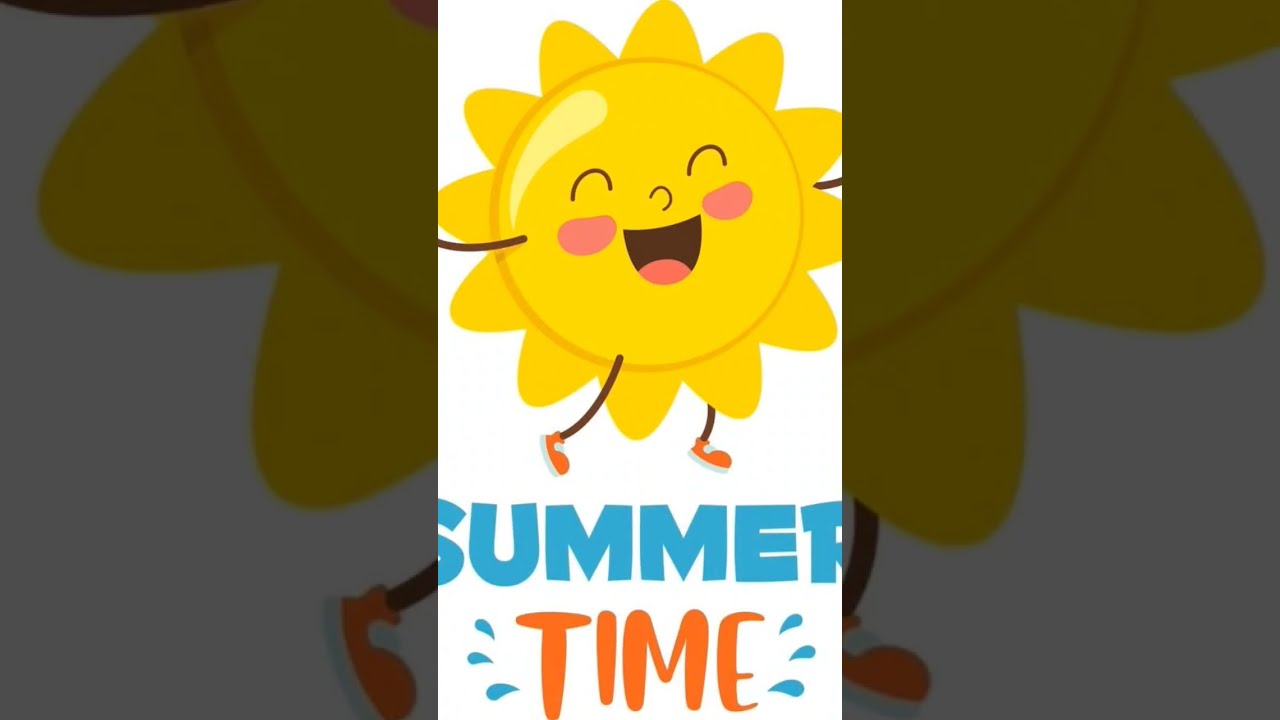The image is a vibrant and playful cartoon illustration of a sun, which serves as a potential thumbnail for a kid-friendly video, possibly on Instagram or TikTok, celebrating summertime. The sun is depicted with a joyful expression—eyes closed in a wide, rosy-cheeked smile, showing a pink tongue and a black open mouth. It has thin, black arms and legs stretching outward and is wearing orange shoes with white laces, giving it a lively, dancing appearance. The background is a simplified, grayed-out version of the main image, adding depth without distraction. The word "summertime" is prominently displayed beneath the sun, with "summer" in blue and "time" in orange, complemented by playful water droplets. The simplistic yet artistic graphic suggests it could be from a children's program, celebrating the joy of summer break.